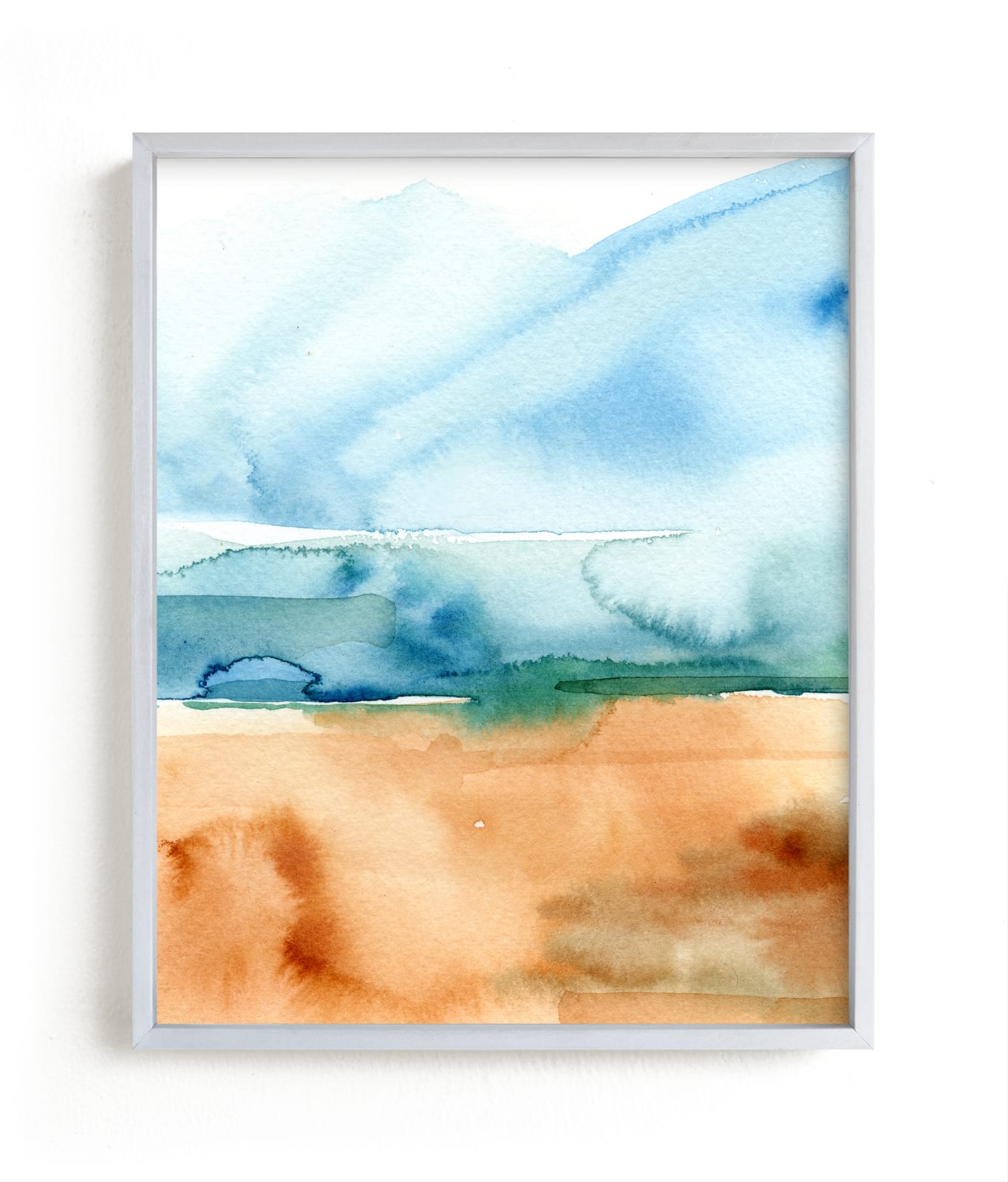This image is a framed, abstract watercolor painting hanging on a wall, enclosed by a gray frame. The painting features a conceptual blend of colors without depicting any concrete objects, emphasizing the fluidity and merging properties of watercolors. 

At the bottom of the painting, there is a section dominated by shades of orange and reddish-browns, interspersed with dark lines that streak through this area. There are also patches of tan and light brown, suggestive of a sandy, earthy texture. Moving upwards, the middle section transitions into various hues of green, representing a grassy or vegetative area, with jagged outlines hinting at natural foliage.

Towards the top, the painting features lighter shades of blue, blending into whites and darker blues, creating an effect reminiscent of a mountainside or sky. The colors bleed into each other, creating a harmonious blend of green and blue tones that suggest a serene, natural landscape. The image has a faux shadow around the frame, indicating it is being showcased for sale on a website.